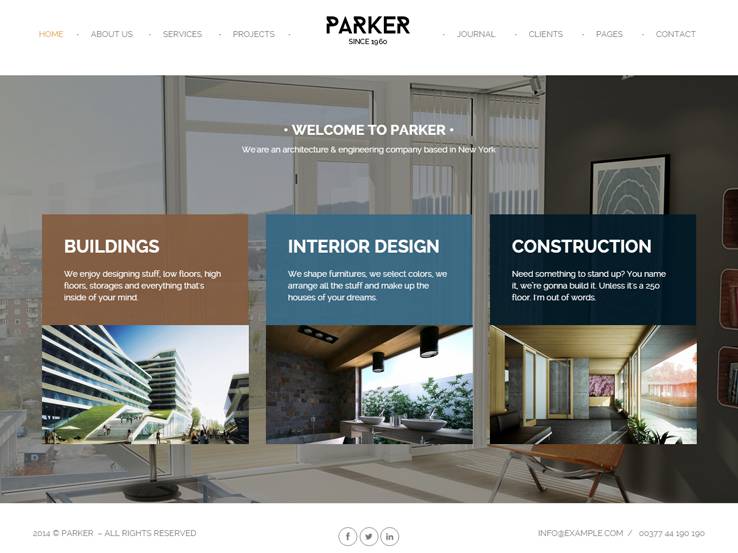Here is a detailed and cleaned-up caption:

---

The screenshot presents the homepage of a website titled "Parker, since 1960." The website's name is prominently displayed at the top in black, bold font. To the left of the name, there are menu selections labeled as Home, About Us, Services, and Projects. To the right, more menu options include Journal, Clients, Pages, and Contact. The Home menu is highlighted, indicating the current screen view. 

Below the navigation bar, an introductory section welcomes visitors with the statement: "Welcome to Parker. We are an architecture and engineering company based in New York." This section is accompanied by a picture depicting the interior of what appears to be an office space.

Further down, the homepage features three interactive options under a set of categories: Building, Interior Design, and Construction:

1. **Building:** Described with a message that reflects their enthusiasm for designing various structures, including low and high-rise buildings, storages, and customized interiors based on client imagination.
2. **Interior Design:** Emphasizes their expertise in shaping furniture, selecting colors, arranging items, and creating dream homes.
3. **Construction:** Highlights their capability to build bespoke structures, mentioning their flexibility unless it involves an impractically tall building, humorously ending with "Unless it's a 250 floor, I'm out of words."

Although the descriptions in the boxes are somewhat informal, they provide a glimpse into the services offered by the company.